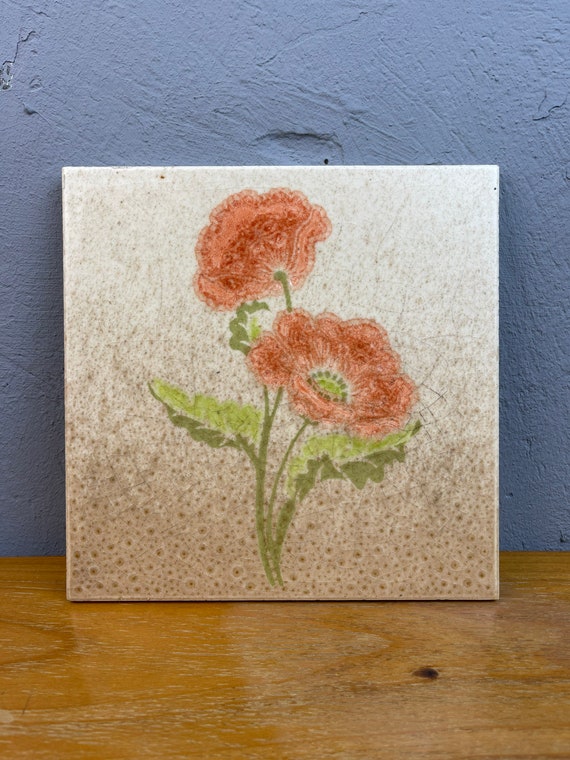The photograph features a square white canvas tile resting atop a honey-gold hardwood table, positioned against a blue stucco plaster wall. The painting on the canvas depicts a plant with two vivid red flowers. The larger blossom is angled toward the right center, fully open with reddish-pink petals encircling a green bud, while the smaller blossom at the top faces away, showing its red-interior petals from below. The flowers are connected by green stems, one curving gracefully downwards. At the base of the stems are light green leaves, which transition to darker green on the shadowed side, including a smaller leaf further up the stem. The lower part of the canvas shows a dense cluster of red speckles, which gradually lighten and thin out toward the top, revealing more of the white background.